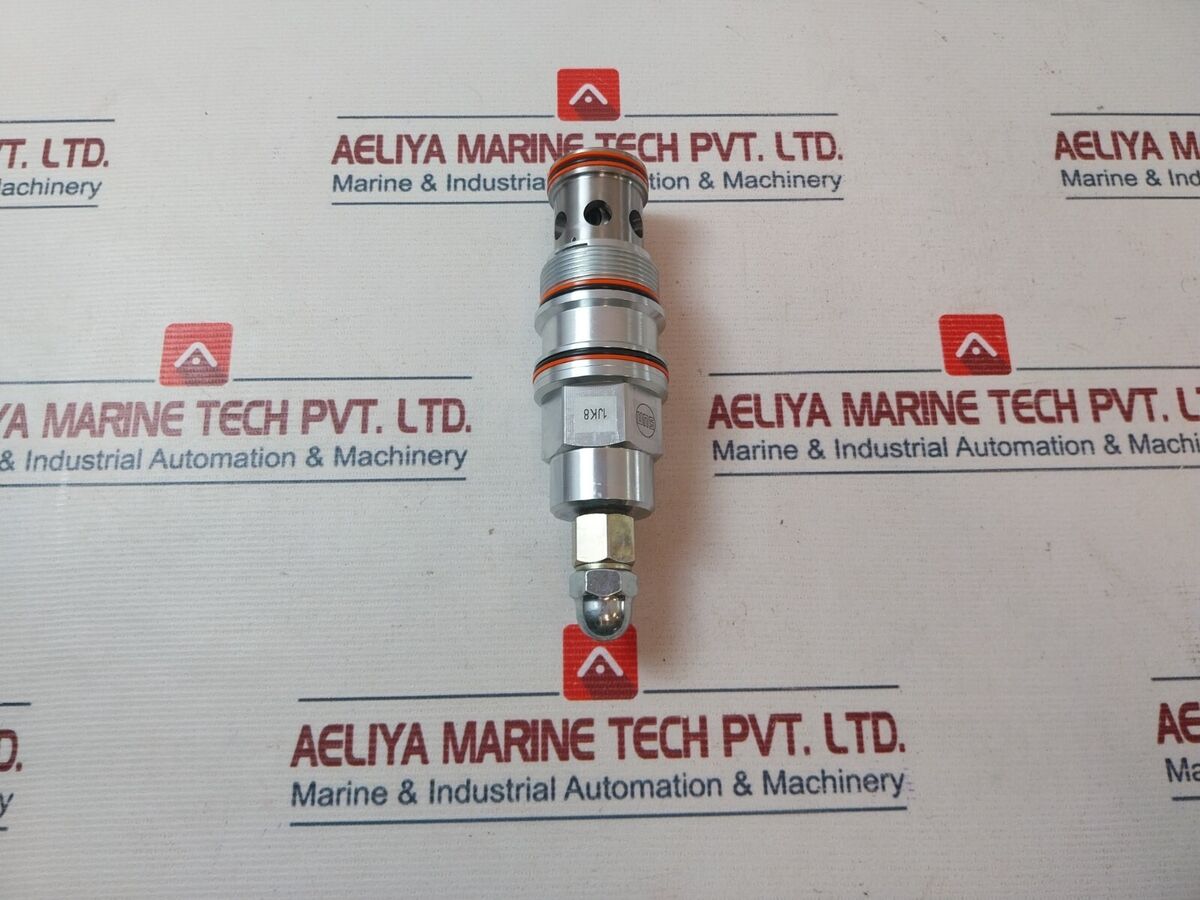The photograph features a detailed image of a cylindrical metal component, possibly a fuel injector or sparking device, characterized by its threaded ends and ports presumed for fuel and air mixture delivery. It has a covering nut likely for a fuel line connection and an upside-down label reading "1JK8" on a white square. The metal piece is predominantly silver, with a couple of rings in orange and black encircling it, creating a prominent visual detail. The image is set against an off-white or white background that appears to be some form of printed cardboard, repeating the company text and logo. The text in red reads "AELIYA Marine Tech PVT Ltd," while "Marine and Industrial Automation and Machinery" is written beneath it in blue. Above the text, there is a small square logo featuring a stylized white arrow with a circular dot head, likened to a modified birdhouse on a maroon background. Additionally, a smaller red box with a caveat 'TP' symbol and dot lies above where the company name is printed. The entire composition suggests the metal part is associated with marine industrial applications, with a striking mix of professional branding and technical hardware.